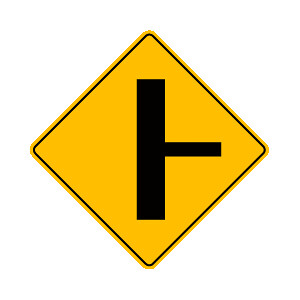This image features a digitally recreated or pre-print photo of a yellow road sign, designed to appear as a square turned on its side, forming a diamond shape. The sign is perfectly symmetrical with a slight black border running along its edges. In the center of the sign, a bold black vertical line extends from top to bottom, representing a main road. A smaller horizontal black line intersects this vertical line from the right, indicating the presence of a side road. The sign, often mounted on highways or streets, serves as a warning to drivers about an upcoming three-way intersection, allowing them to anticipate potential traffic merging from the side road. The photograph, against a white background, highlights the clear and distinct features of the sign, emphasizing its function as a critical traffic safety indicator.